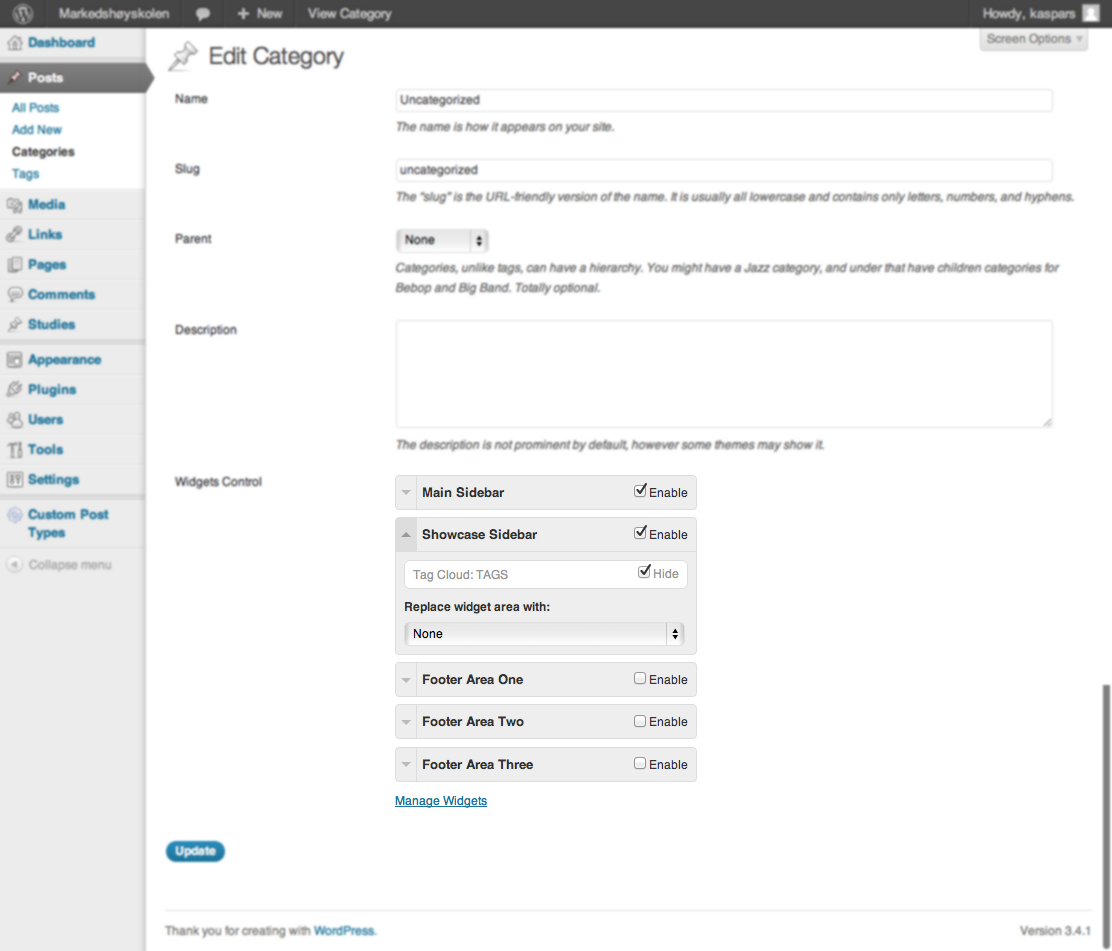The image depicts a user interface of a website's content management system. At the very top, a grey banner spans the full width of the screen, displaying the website's logo and name prominently. On the left side of this banner are buttons for creating new content and viewing categories. Towards the far right of the banner is a login button.

On the left-hand side of the interface, a vertical menu lists various options, each labeled with different functionalities such as Dashboard, Posts, Categories, Tags, Media, Links, Pages, Comments, and Studies. These categories further subdivide into more specific options; for instance, 'Posts' is expanded into 'All Posts', 'Add New', and 'Categories', while 'Categories' includes additional sections like 'Tags', 'Media', and 'Links'. Lower in the menu, additional sections appear, including Appearance, Plugins, Users, Tools, Settings, and Custom Post Types.

The 'Categories' option is highlighted in black, indicating it is currently selected. The right side of the screen displays the 'Edit Category' page. Here, several fields are available for editing details about categories. The first field is labeled 'Name', featuring an input box for the category name. The next field, labeled 'Slug', also has an input box, although the term "slug" might seem unconventional. Following this is the 'Parent' field, which has a default value of 'None' and can be adjusted to set a hierarchical relationship between categories. The 'Description' field is a large text area, allowing for a substantial amount of text to be entered. 

At the bottom of this section are widget controls, providing a variety of settings for managing different sidebars and widgets, such as the main sidebar, additional sidebars, showcase sidebars, and other widget areas designated for figures and additional content zones.